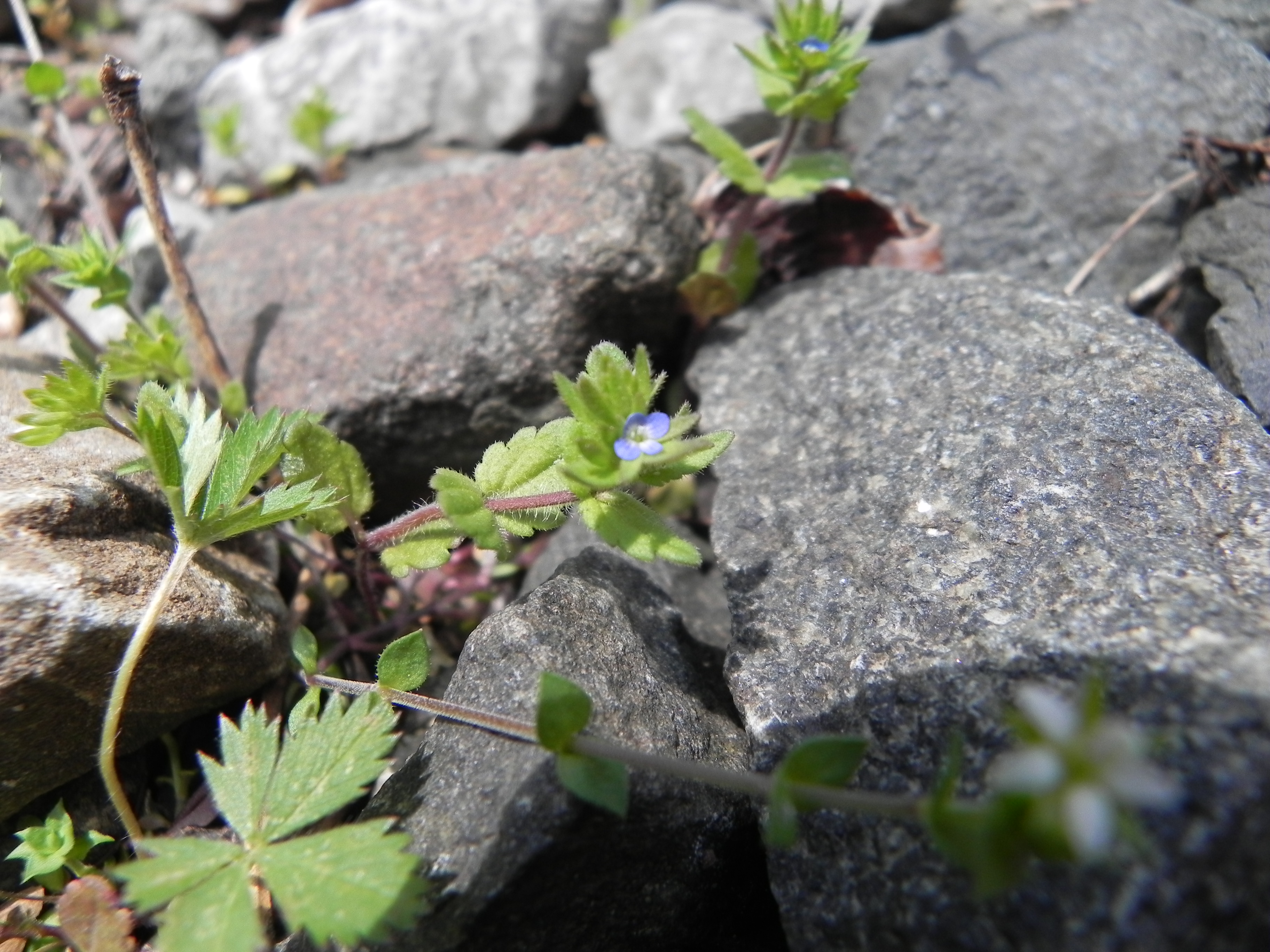This outdoor daytime photograph captures a vivid scene of wild, strawberry-like plants growing amidst a collection of varied gray rocks. The image, approximately 6 inches wide and 4 inches high, is taken from an overhead perspective, focusing sharply on the foreground details including the individual characteristics of the green leaves and the slightly hairy stems. The rocks range in color from deep gray, some speckled with lighter gray spots, to gray stones with reddish accents and even hints of pink and white. Central to the image are three flowers with striking blue petals and white centers, and additional smaller white five-petaled flowers are also visible. The plants, bearing a close resemblance to strawberries typically found growing on the ground, emerge robustly between the rocks, sporting leaves that align closely with those of strawberry plants. The sharpness of the photograph allows for an appreciation of the textures and colors in the foreground, while details in the background become more blurred. Sunlight bathes most of the scene, though the lower right-hand corner falls into shadow, enhancing the contrast and depth of the image.